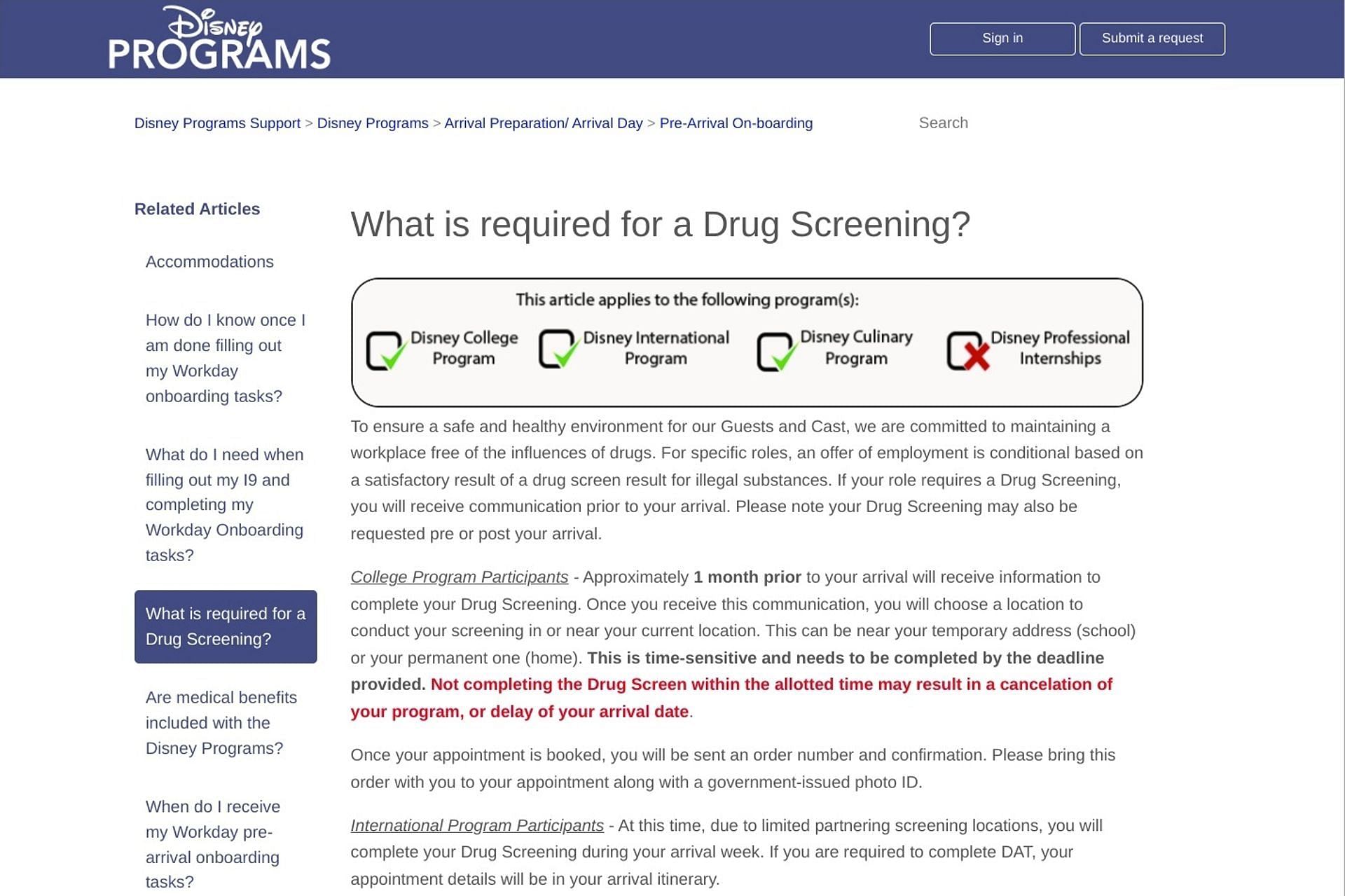Screenshot of the Disney Programs Support Page

The screenshot displays the Disney Programs Support interface, specifically focusing on the various options and helpful articles available for program participants. The main sections visible include:

- **Disney Program Sign In**
- **Submit a Request**

Highlighted is a navigation menu option backed by a purple rectangle, indicating it is currently selected. The options listed under this selected section include:

- **Arrival Preparation**
- **Arrival Day**
- **Pre-Arrival Onboarding**
- **Search**

Several related articles are also visible, covering topics such as:

- **Accommodations**
- **How do I know once I am done filling out my Workday onboarding tasks?**
- **What do I need when filling out my I-9 and completing my Workday onboarding tasks?**
- **What is required for a drug screening?**
- **Are medical benefits included with the Disney Programs?**
- **When do I receive my Workday pre-arrival onboarding tasks?**

The article in question, which is highlighted, addresses the requirements for drug screenings within Disney Programs. It explicitly states:

"To ensure a safe and healthy environment for our guests and cast, we are committed to maintaining a workplace free of the influence of drugs."

Additionally, the article is applicable to the following programs, with status indicated by checks and an 'x':

- Disney College Program ✔
- Disney International Program ✔
- Disney Culinary Program ✔
- Disney Professional Internships ✘

The page provides extensive information to ensure readiness and compliance for incoming program participants, reflecting Disney's commitment to safety and clinical standards.